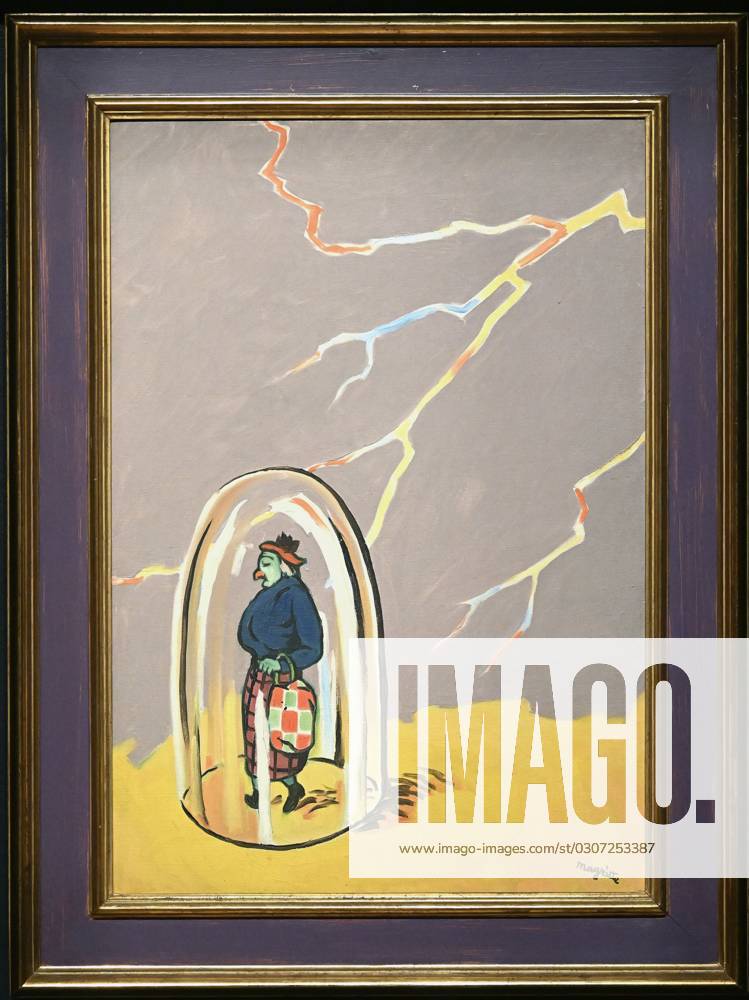The image depicts a detailed painting within a multi-layered frame. The outermost framing is a combination of black and gold, which encloses a purple backdrop. Inside this is another gold trim, framing a rectangle that adds further depth to the composition. In the center of the painting is a fantastical figure—a woman with blue skin and a green, beak-like feature resembling a bird. She is attired in a blue jacket, plaid pants, and is carrying a green and red checkered bag. The woman appears to be immobilized, trapped under an upside-down glass dome. She stands on a yellow floor with a gray backdrop behind her. Surrounding her, vibrant lightning strikes in colors of orange, white, yellow, and blue crisscross the scene. The bottom right corner of the painting bears a watermark reading "Imago" along with a link to the image.